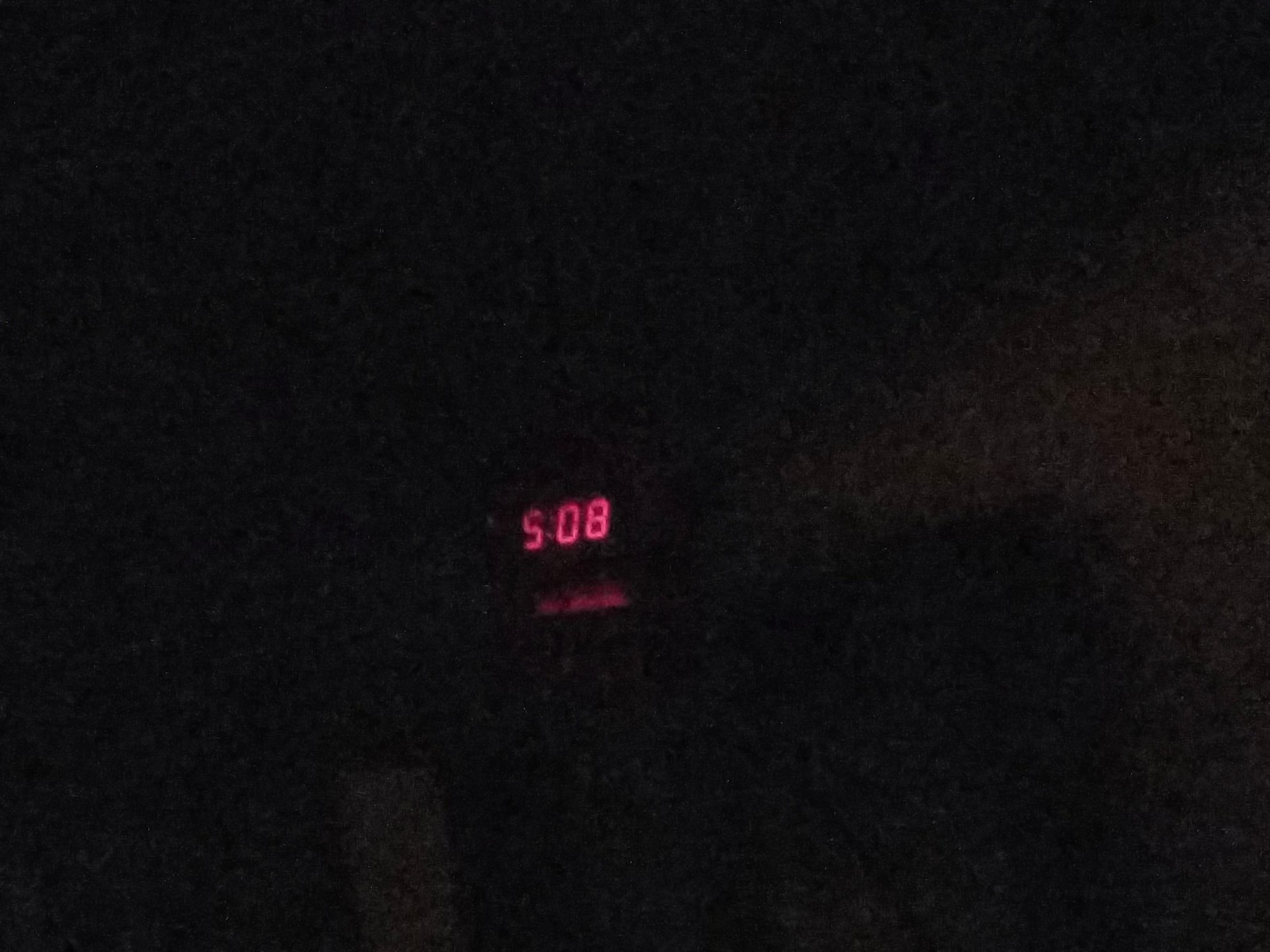This color photograph is extremely dark and blotchy, making it challenging to discern details. The background predominantly features deep black, especially concentrated in the upper left corner and central areas. Towards the bottom of the image, faint grey shadows emerge, adding slight variations to the darkness. Central to the composition is a discernible blocky shadow, with another lighter blocky shadow positioned near the right edge. A key element of the photograph is positioned centrally—a set of fluorescent numbers glowing in a bright red, resembling the display of a digital clock. The digits read "508." Beneath this display, a partial, thin linear reflection is visible, suggesting that the clock is placed on a reflective surface. Other details in the photo remain obscure due to the pervasive darkness and blotchiness.